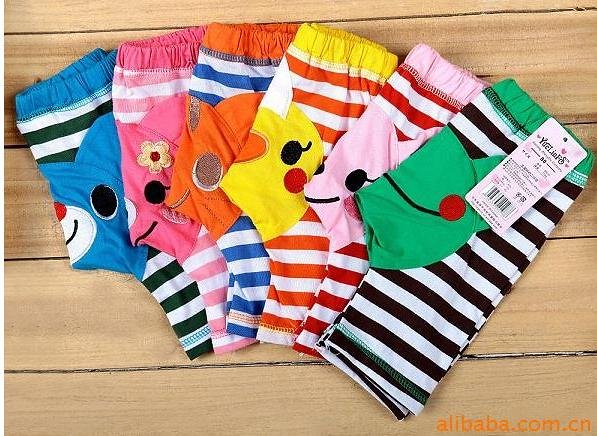The image features an assortment of six pairs of very colorful and small children's shorts or swim shorts, each with a striped design and a cute animal face on the back. The shorts are arranged in a fan-like pattern on a wooden surface, likely showcasing their designs for display purposes. From left to right, the first pair is blue with green stripes, featuring a smiling blue bear with black eyes. Next is a pink pair adorned with a little bunny rabbit and a golden flower by its ear. The third pair is orange and blue striped, displaying an orange creature of unspecified type. The fourth pair is orange and yellow, with a chicken sporting red cheeks and an orange beak. The fifth pair combines red and pink stripes with what looks like a bunny, and the final pair has black stripes with a green waistline featuring a frog. Each pair has a colorful, striped design and an animal's face on the butt area. Additionally, one pair has a tag with a barcode, and the bottom right corner of the image includes the website "alibaba.com.cn".